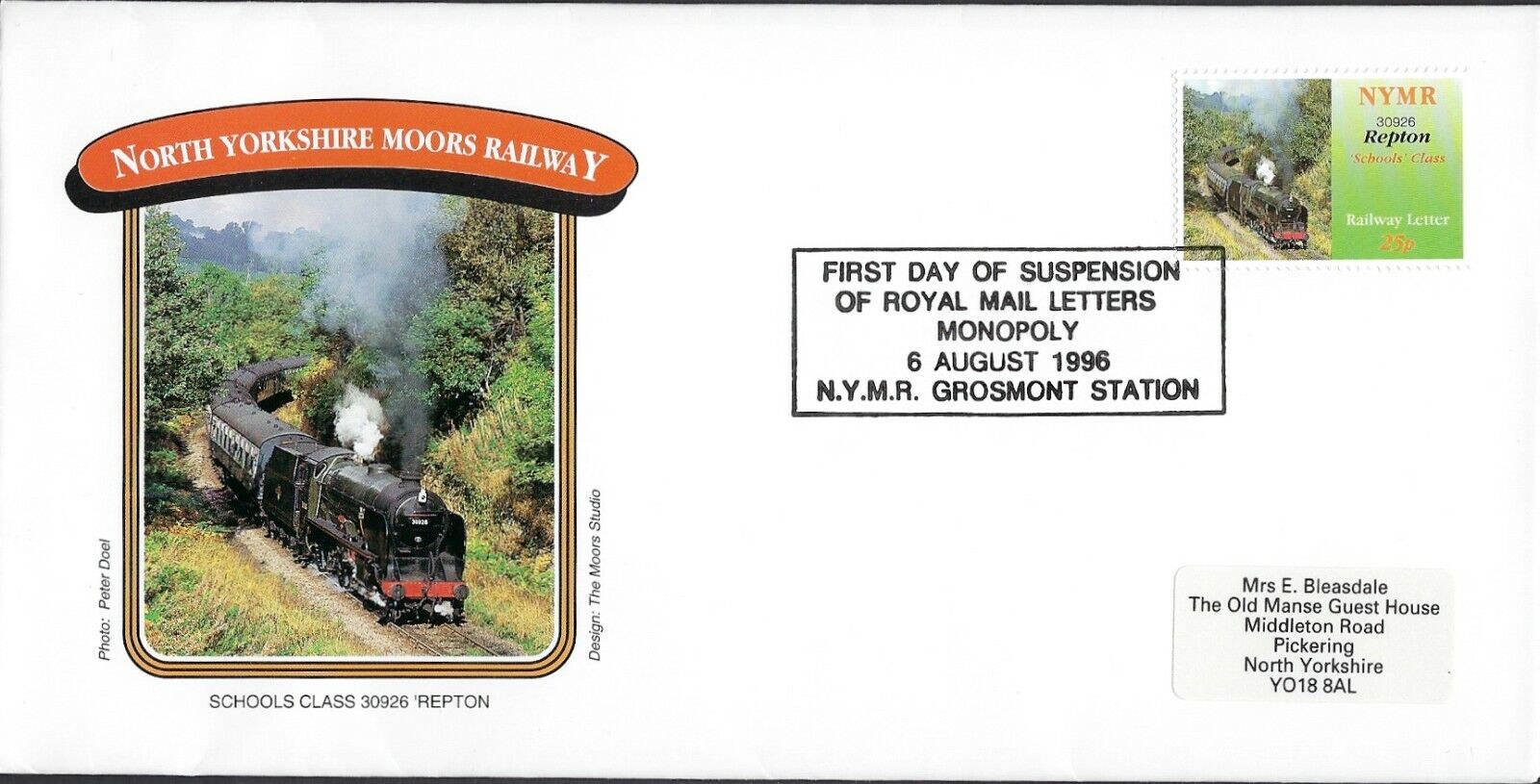This postcard from the North Yorkshire Moors Railway showcases a striking photograph by Peter Dole, depicting a black steam locomotive with a red bumper, identified as Schools Class 30926 Repton. The train is captured winding through a scenic mountain pass, framed beautifully by lush trees. The postcard, designed by The Moors Studio, features a special North Yorkshire Moors Railway stamp in the upper right corner with the same train image, marked NYMR. The postcard bears a noteworthy stamped seal commemorating the First Day of Suspension of Royal Mail Letters Monopoly on 6 August 1996, at NYMR Grosmont Station. In the bottom right corner, a typed address reads: Mrs. E. Bleasdale, The Old Manse Guesthouse, Middleton Road, Pickering, North Yorkshire, YO18 8AL.